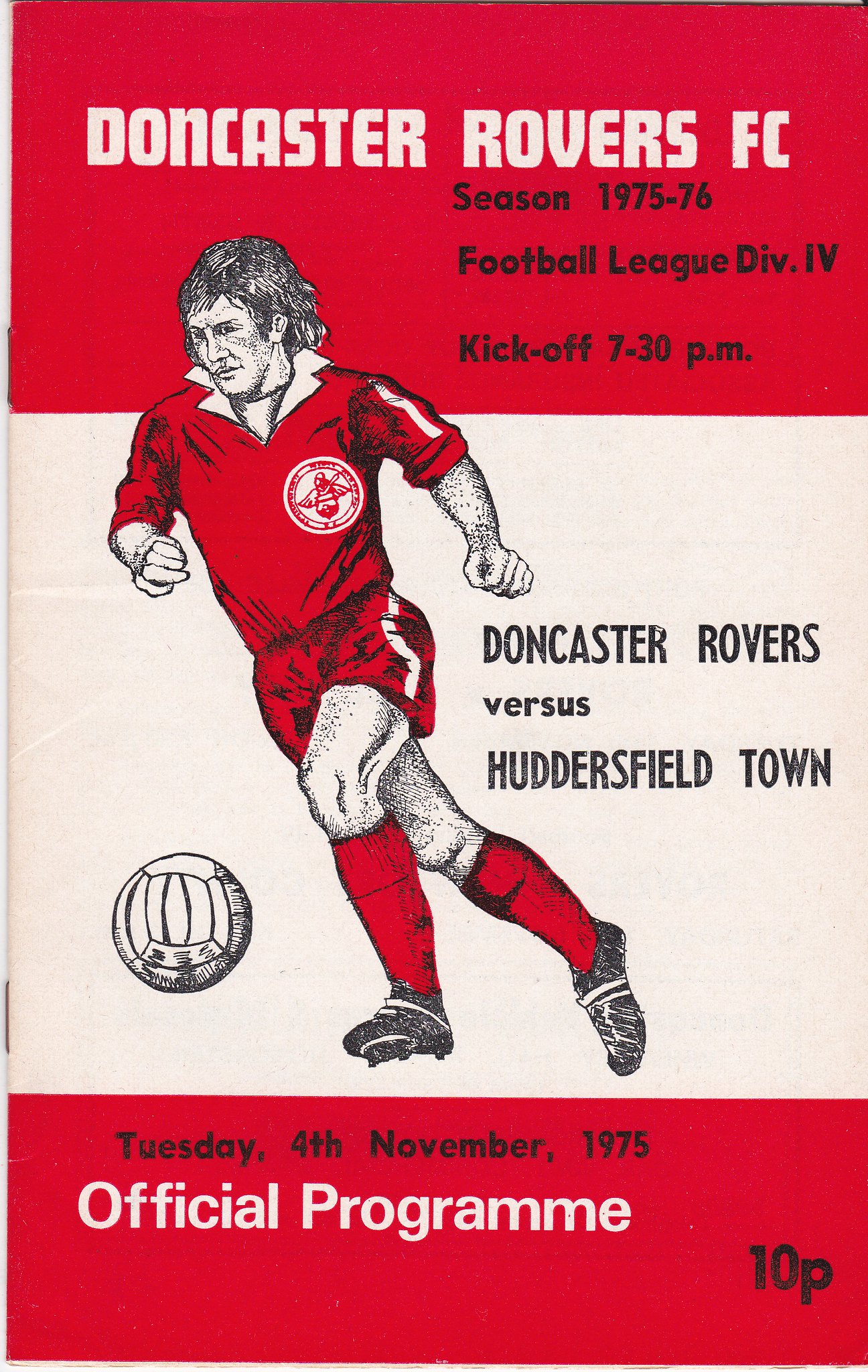This vintage advertisement, from the 1975-76 season of Football League Division 4, features a bold red header with "DONCASTER ROVERS FC" prominently displayed in all caps, using a striking white font against the vibrant background. Beneath this, on the right side, crucial match details are listed in black font, indicating the season and the kickoff time of 7:30 pm. Centrally positioned, a white box contains an intricate sketch of a footballer dressed in a red outfit, dynamically engaged in kicking a soccer ball. To the right of this illustration, "Doncaster Rovers vs. Huddersfield Town" is printed in black, drawing focus to the competing teams. The advertisement's lower portion features a smaller red box, which in black font, announces the date as Tuesday, 4th November 1975. Below, in larger white text, the phrase "Official Programme" is spelled out, notably ending with an additional 'E'. Lastly, the bottom right corner indicates the price, "10 pence", again in black font.